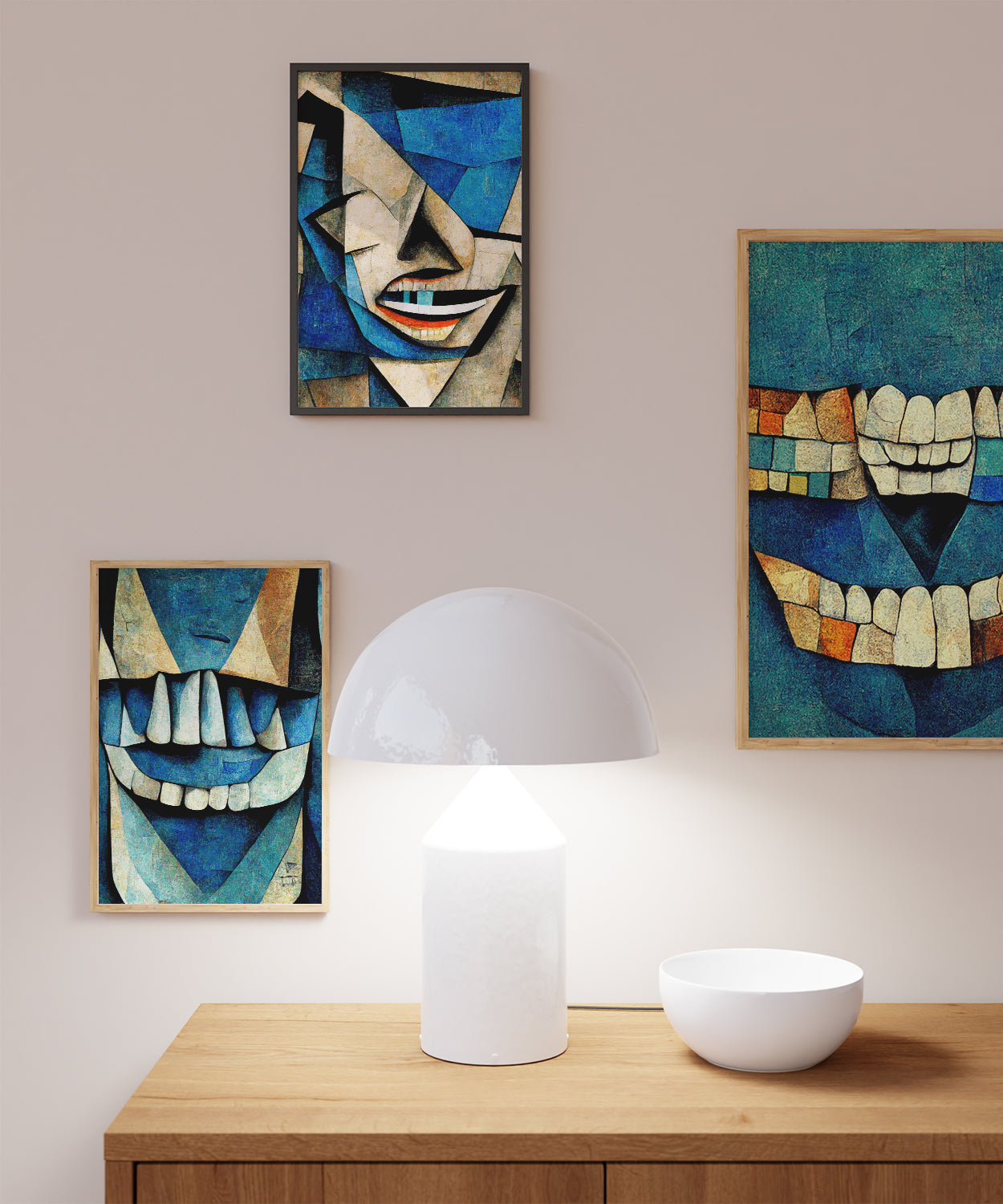Against a light purple background, three abstract paintings adorn the wall, each in a distinct yet cohesive style reminiscent of Cubism or Picasso. The dominant hues across the paintings are blue, beige, black, and white, with pops of red, orange, and yellow. The largest painting on the right captures abstract teeth shapes—white at the center, transitioning to beige, brown, and blue at the edges—set against a predominantly blue backdrop. The top-left painting showcases abstract forms suggesting a mouth with red lips, where blue, beige, black, and white intermingle. Below it, the bottom-left painting mirrors these color motifs with blue, black, and beige composing yet another abstract set of teeth. Each painting is framed in thin wood, with the top one in a dark gray frame and the others in natural wood tones.

Below the artwork, a light wooden table supports a modern white lamp with a white lampshade and a white bowl next to it, providing an elegant touch to the space. The clean lines and contemporary feel of the table and lamp complement the striking, abstract nature of the art above.